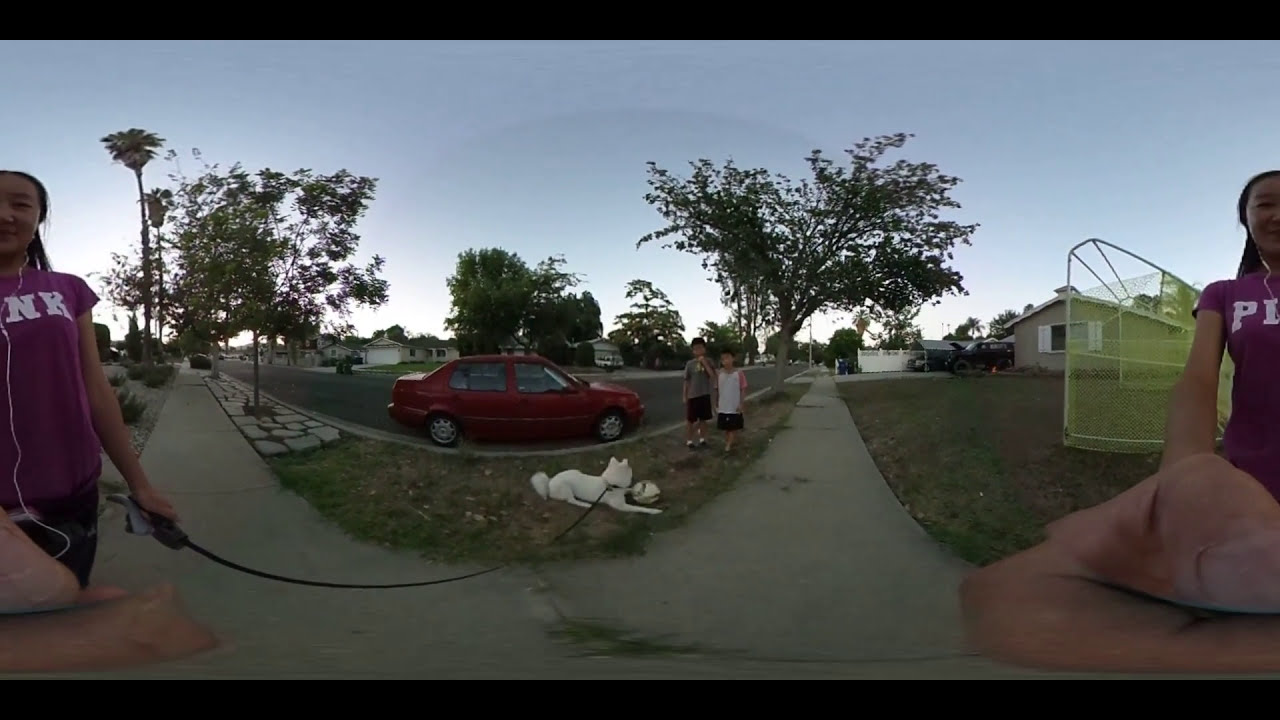In this distorted fisheye lens photograph, a bustling sidewalk scene unfolds in a light gray path bordered by lush green grass. This sidewalk extends from the background to the foreground, flanked on either side by vivid, dynamic elements. On the left, a young boy dressed in a white shirt with black shorts, and another boy in a gray shirt with black shorts, both with dark hair, stand on the grass near the street. Between them, a white dog with a black leash lies on the grass, its eyes fixed attentively on the children. A red car is visible near them, and a tall tree with dense green foliage provides a natural backdrop.

The dog plays a central role, connected by its leash to a girl who appears twice in the image due to the fisheye effect. She is dressed in a purple shirt emblazoned with the letters "N" and "K" in white, and black shorts. Her black hair is pulled back, and on the right side of the image, her large, outstretched hand further distorts the scene, with additional letters "P" and "I" visible on her shirt. Behind her, a yellow barrier made of expanded metal separates the scene from a light brown house with white window panes and an arched roof.

In the background, mixed tree varieties, including pop trees and deciduous trees, contribute to the natural ambiance. The sky, with its subtly gray hue, casts a serene light over the vibrant scenario, where both mirrored and original elements create a kaleidoscope-like effect. To the right, near the girl, an ambiguous structure resembling a white pole and netting—possibly part of sports equipment or a fence—adds to the image's complexity. Amidst this captivating array, the image captures a moment of everyday activity frozen in a kaleidoscopic lens.